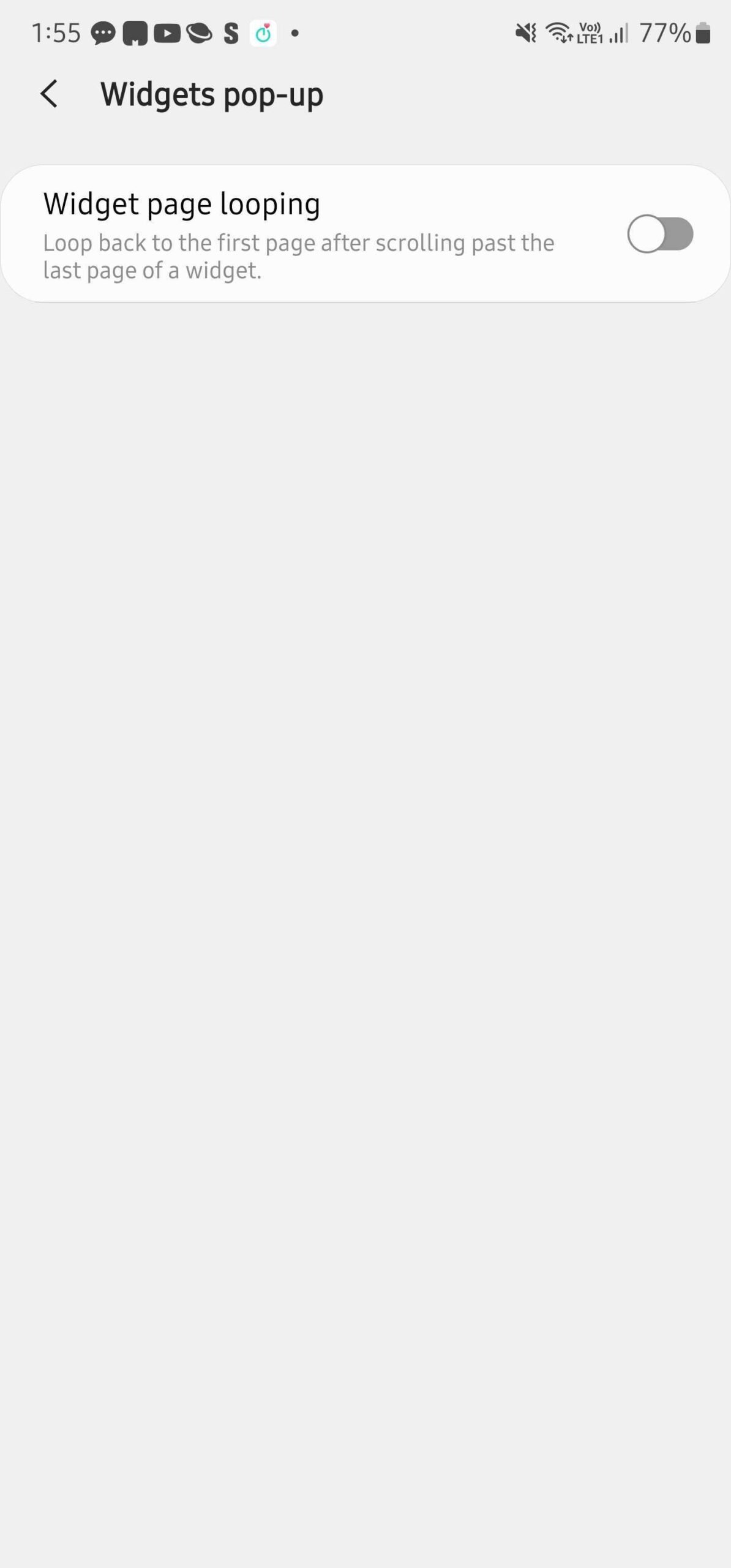The image is a screenshot of a smartphone display. The visible elements include a messaging app, an internet browser, and an icon featuring a square with a wedge cut out at the bottom. Importantly, the status bar at the top shows a battery level of 77% and indicates that the signal strength is adequate. The brand "Samsung" is also mentioned within the image. The entire interface is set against a gray background.

Additionally, there is an arrow pointing to the left, accompanied by bold text that reads "Widgets pop up." Below this is a small, white rectangular box containing the text "Widget page looping," which describes a feature to loop back to the first page after scrolling past the last page of a widget. To the side, there's an option to toggle this feature on or off, which is currently set to off. The rest of the image maintains a consistent gray background.